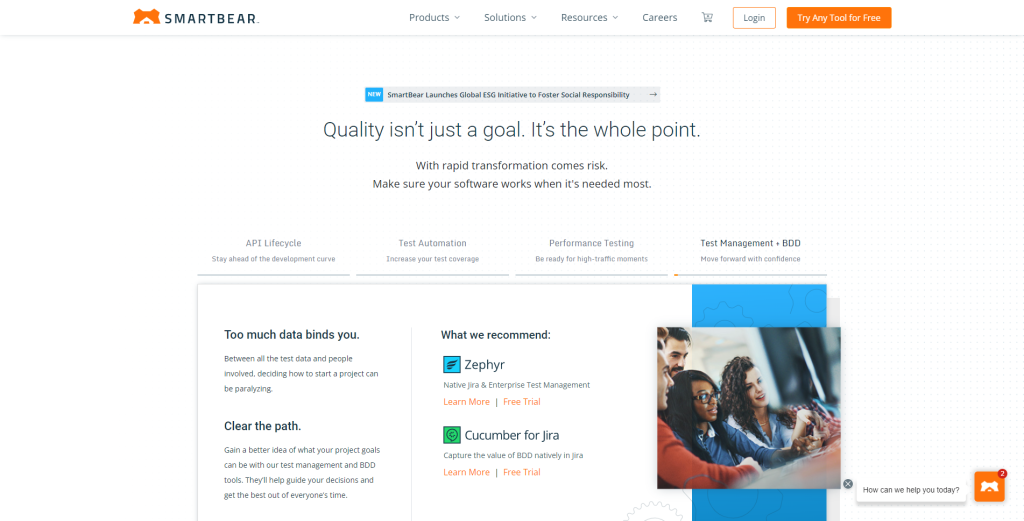Landing page design for SmartBear:

At the top of the page, there's a menu bar with a sleek black and white background. The menu includes tabs labeled "Products," "Solutions," "Resources," and "Careers." On the far right of the menu bar, there is a "Login" button followed by a "Try Any Test for Free" button.

Beneath the menu, there's a prominent header in black text on a white background that states: "Quality isn't just a goal, it's the whole point." Just below this, a subheading reads: "With rapid transformation comes risk. Make sure your software works when it's needed most."

Further down, several small menu headings are listed in a row, including "API Lifecycle," "Performance Testing," and "Test Management," though the text is quite small and somewhat difficult to read.

Towards the bottom, within a gray outlined box with a white background, there's an image on the far right depicting four individuals in an office setting, looking intently at something off-screen. To the left of this image, there are descriptive texts providing further information about the company’s offerings and value propositions.